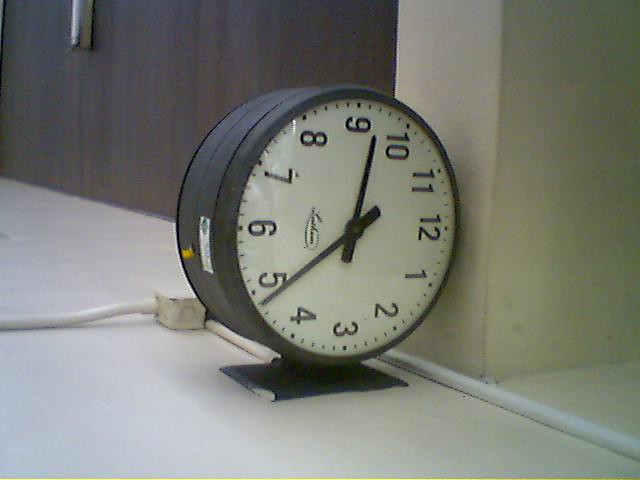In this visually intriguing scene, a dark gray wall forms the backdrop for a composition of striking elements. Attached to the wall is a long, white object, its simplicity contrasting against the darker hue. The floor, in a light gray shade, complements the wall and provides a neutral base for the main feature: a large clock. This clock, with a dark gray frame and a small stand, is notably placed on its side. Its white face is adorned with black, regular numerals and matching black hands, though its orientation is unconventional – the numerals nine and three occupy the vertical axis, while twelve and six are positioned horizontally, creating an intriguing visual shift. A thick, white electric cord lies beneath the clock, contributing to the scene's modern and somewhat abstract feel. In the background, part of a light gray wall and a thin white strip add layers to the composition, enhancing the depth and complexity of the setting.